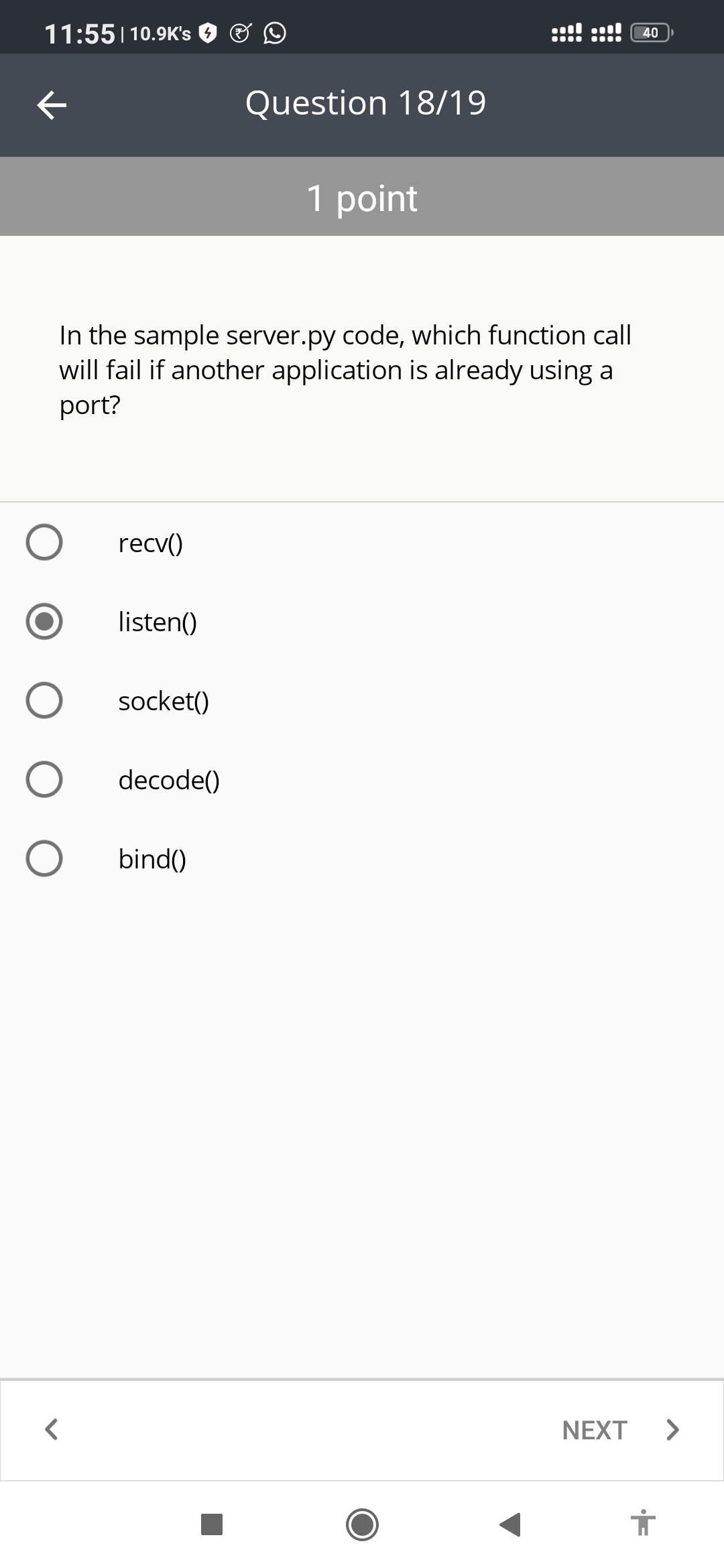This is a detailed screenshot of a cell phone screen, illustrating a question from a server programming quiz and the phone's status bar. 

**Status Bar:** 
At the very top, a black bar displays in white lettering and icons the time "11:55". Next to it is a pipe symbol, "10.9 KBs", a white shield icon with a black lightning bolt in it, a gray circle with an indiscernible white squiggle, a white text bubble with a diagonal phone receiver inside, four filled white bars, and a battery icon indicating "40%" remaining.

**Gray Bar:**
Below this, on a dark gray bar, a white backward arrow appears on the left. Centered on the same bar, it reads "Question 18/19" indicating the current quiz question out of a possible 19. 

**Light Gray Bar:**
Directly under this, a light gray bar has "1 point" written in white.

**Question Section:**
Further down, a white section displays the question related to server programming. The text asks: "In this sample server.py code, which function call will fail if another application is already using a port?" Five possible answers are listed below, each accompanied by a radio button on the left:
1. "RECV()" - not selected.
2. "listen()" - selected.
3. "sockets()" - not selected.
4. "decode()" - not selected.
5. "bind()" - not selected.

**Navigation Buttons:**
At the bottom of the screen, there is a left-facing back arrow, the word "Next" in gray with a right-facing arrow, and across a gray bar, four gray icons: a square, a circle, a backward triangle, and a human body shape.